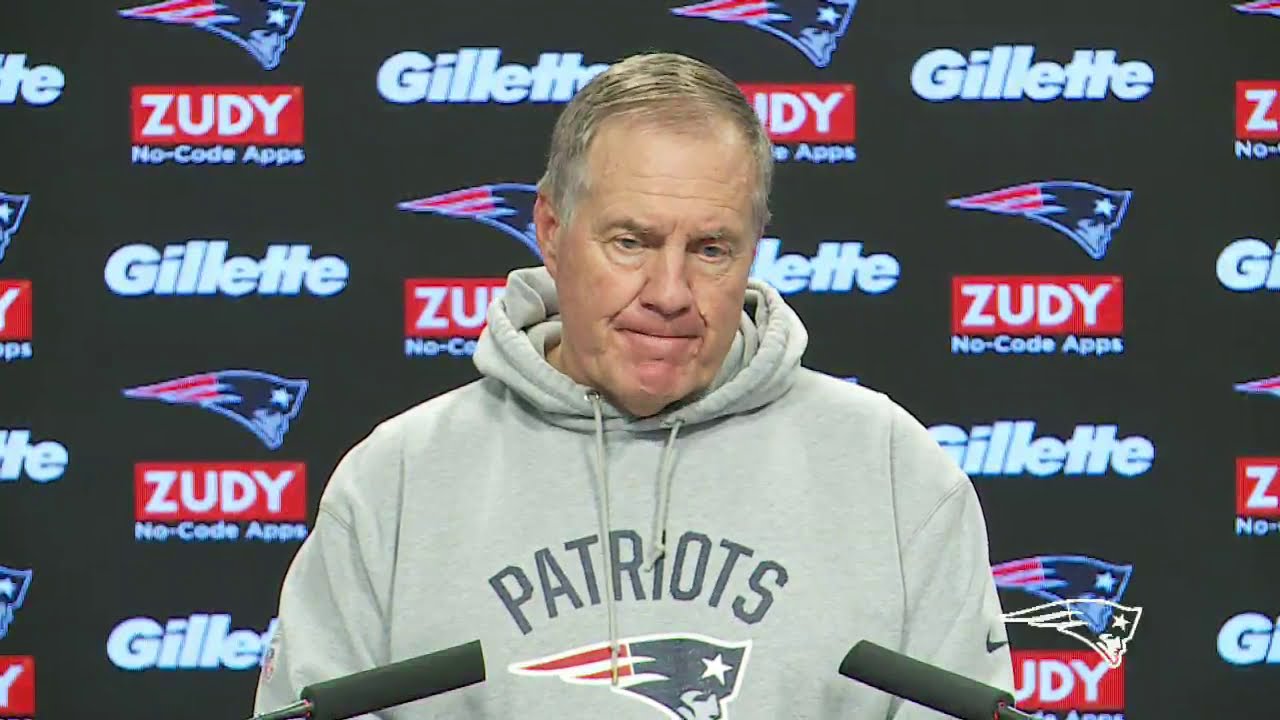The image features an elderly man, approximately 60 to 65 years old, with pale skin, blue eyes, and hair combed over from left to right. He is wearing a gray Patriots hoodie prominently displaying the team's name and logo. Positioned centrally in the image, this man stands before two microphones angled toward his chest, suggesting he is at a press conference, likely discussing his retirement as the coach of the New England Patriots. The background is adorned with a repeating pattern of the Patriots logo accompanied by the names "Gillette" and "Zooty NoCodeApps" as sponsors. The setting appears to be indoors, characterized by a color palette of red, white, blue, tan, gray, and black, consistent with a formal event or post-game press briefing.